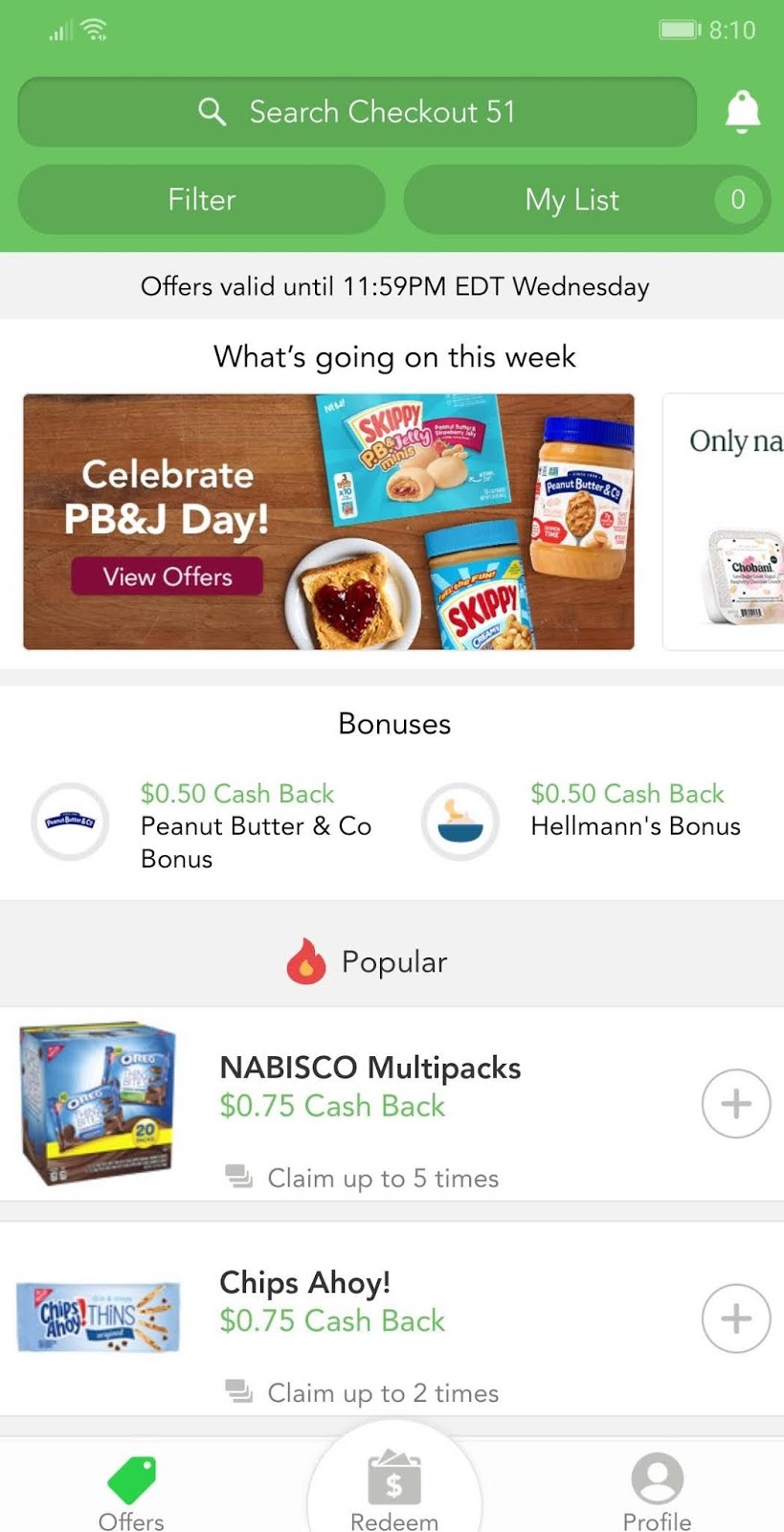This image is a screenshot captured from a smartphone in portrait orientation. The photo is rectangular, and the top features a green horizontal rectangular border. Within this border, the status bar displays the connection strength at 3 out of 5 bars and a fully illuminated Wi-Fi meter. On the top right of the bar, a battery icon indicates that the battery is almost full and shows "810".

Below the status bar, there's a dark green search bar labeled "Search Checkout" in white font, accompanied by a white bell icon on the right. Adjacent to this, there are two text bubbles labeled "Filter" and "My List."

A gray border with black text beneath the bar reads, "Offer is valid until 11:59 EDT Wednesday." Below this text, a section with a white background and black font states, "What's going on this week?"

Following this section, there’s a landscape picture showcasing some peanut butter products with the caption "Celebrate B&J Day." Right underneath, a white box contains a header titled "Bonuses" and details about two cashback offers: "$0.50 cash back on Peanut Butter and Company bonus" and "$0.50 cash back on Hellman's bonus."

Beneath this, another gray border with a flame icon is labeled "Popular," featuring images of products. Specifically, Nabisco Multipacks offer "$0.75 cash back," and Chips Ahoy has a similar "$0.75 cash back" offer.

At the bottom of the screenshot, a green tag labeled "Offers" is prominently displayed. Flanking this tag are two gray icons labeled "Redeem" and "Profile."